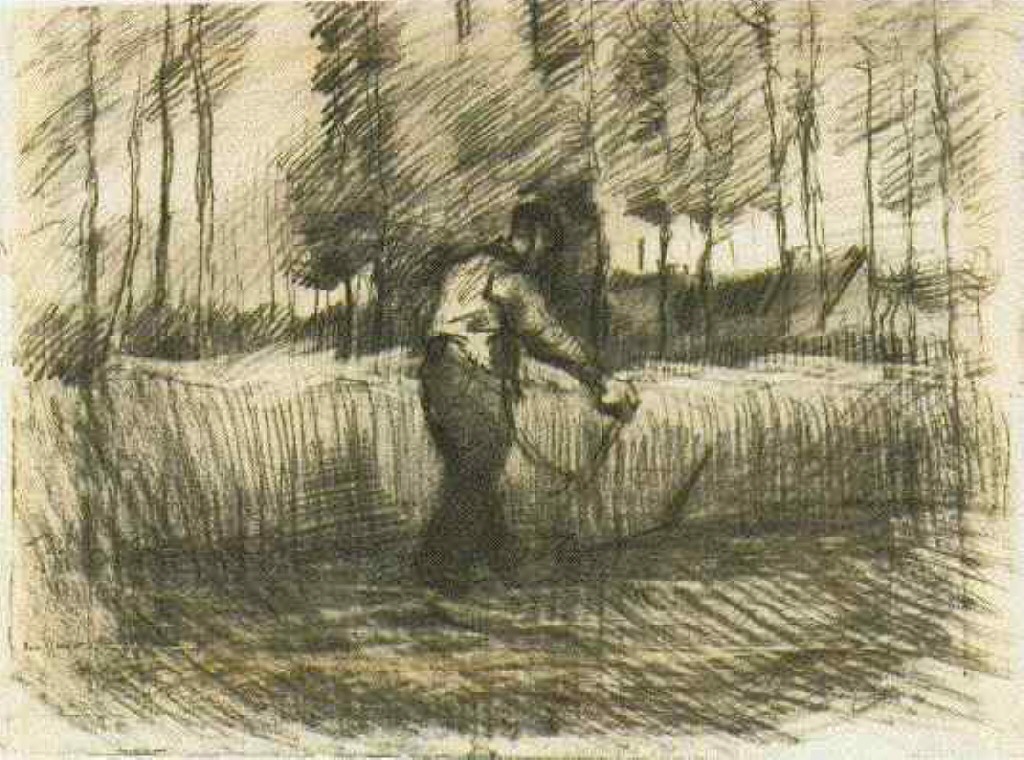In this large, square pen and ink sketch set against a beige background, a man is depicted walking towards the right, framed by a mix of brown and green hues. The sketch uses a combination of back-and-forth strokes to fill in details, giving it a dynamic, textured look. The man, centrally positioned, wears brown pants and a white shirt that appears shaded with brown. His right arm is extended forward, hand open, as if reaching out to grasp something. His head appears bowed slightly, suggesting intent focus, though facial details are indistinct. The figure could be engaged in plowing or trimming hedges, with the suggestion of a plow-like tool in his extended hands.

The ground beneath him is intricately detailed with brown, vertical lines and scribbled textures, creating an impression of shallow water while also resembling uncut grass or wheat. Above, the artwork transitions into a depiction of various trees and bushes, with thin, bare trunks interspersed with vertical lines and zigzag patterns representing leaves, contributing to the scene’s rustic and somewhat wild character. On the left and right edges, thin, poorly developed trees contrast against more robust and leafy counterparts situated towards the center-right. These elements cast dark, shadowy highlights, adding depth and contrast to the overall composition. The bright sky reinforces the daytime setting, devoid of celestial objects, and completes the pastoral, yet sketch-heavy portrayal of the landscape.